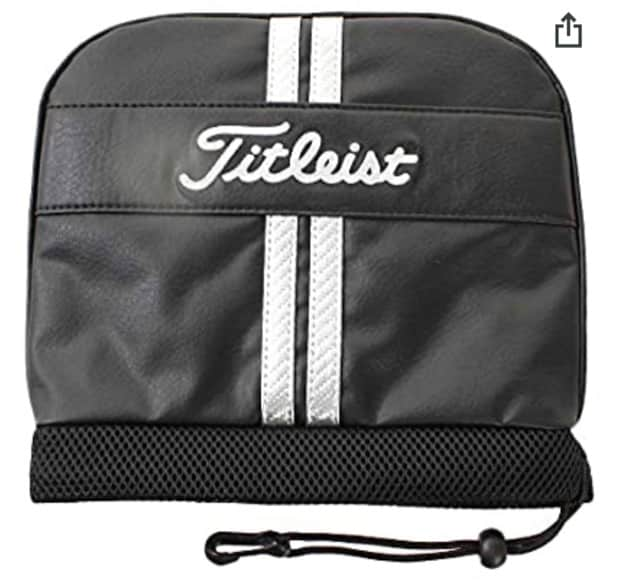The image depicts a centrally positioned Titleist golf bag against a white background. The bag is predominantly black with two vertical white stripes running from the top to the bottom. The brand name "Titleist," written in cursive, appears prominently on the bag. At the bottom of the bag, there is a strap equipped with a hook and loop closure, featuring a grid-like pattern sewn onto it. Additionally, a long string with a bead attached runs from the bottom left of the bag. In the upper right corner of the image, there is a blue square icon with a black upward-pointing arrow, suggestive of a sharing option.